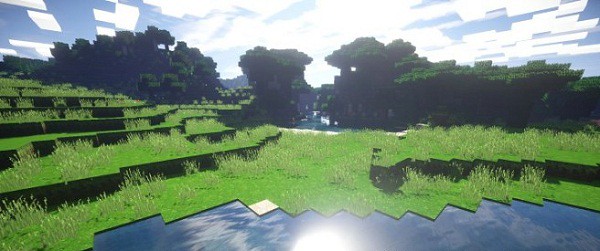This high-quality, computer-generated image appears to be from the video game Minecraft, depicting a vibrant, pixelated landscape. At the bottom of the image lies a shimmering body of water reflecting the sky above. Above the water, the terrain transitions into grassy plains with various patches of tall grass. The right side features progressively higher levels, rising in a stair-like fashion. On the left, a stepped hill ascends six blocks upward. In the background, dense clusters of trees with brown trunks and green, block-like foliage dot the horizon. The sky is adorned with a mix of blue hues and white cubic clouds, whose reflections can be seen in the water below. The overall composition emphasizes the characteristic blocky aesthetics of the game's environment.